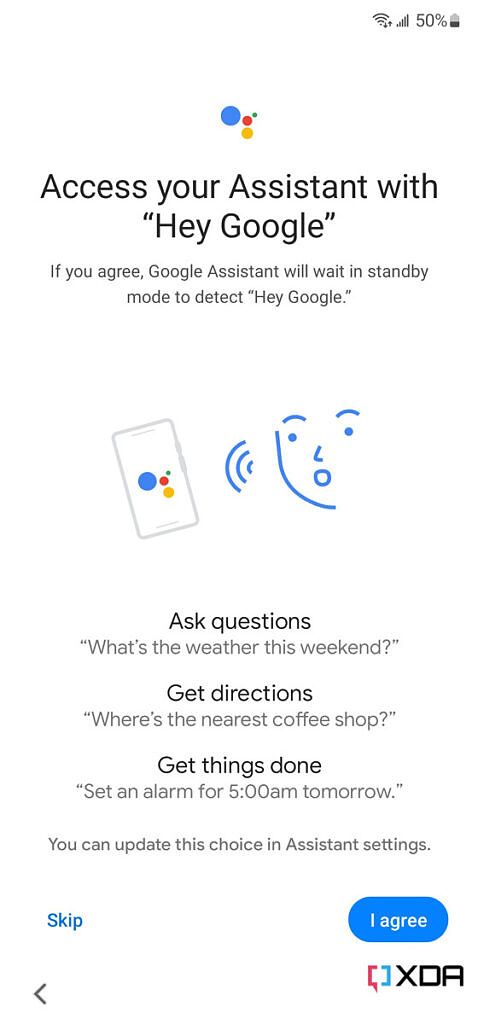In this screenshot demonstrating how to use Google Assistant, a rich array of details is visible. At the top right corner of a white interface, there's a Wi-Fi icon and a data icon, followed by a 50% battery indicator with a half-filled battery icon to signify battery life. Below this, the iconic Google Assistant dots—green, red, yellow, and blue—are prominently displayed, symbolizing the Google Assistant interface.

The screen headline reads, "Access your Assistant with Hey Google." The text explains that if the user agrees, Google Assistant will enter standby mode, actively listening for the "Hey Google" wake command. An illustration showing a face with sound lines emanating towards a phone accompanies this description.

Below the visual, the text lists examples of tasks that can be performed with Google Assistant: "Ask questions: What's the weather this weekend?", "Get directions: Where's the nearest coffee shop?", and "Get things done: Set an alarm for 5 a.m. tomorrow."

Users are informed they can change their settings at any time in the Assistant settings. At the bottom of the screen, two interactive buttons are presented: a blue "Skip" button and a blue "I agree" button with white text, indicating user consent.

Additionally, a back arrow is placed in the bottom left corner for navigation purposes, while at the bottom right a distinctive red and purple icon is featured next to the bold black letters "XDA." The exact meaning of "XDA" isn't clarified in the screenshot.